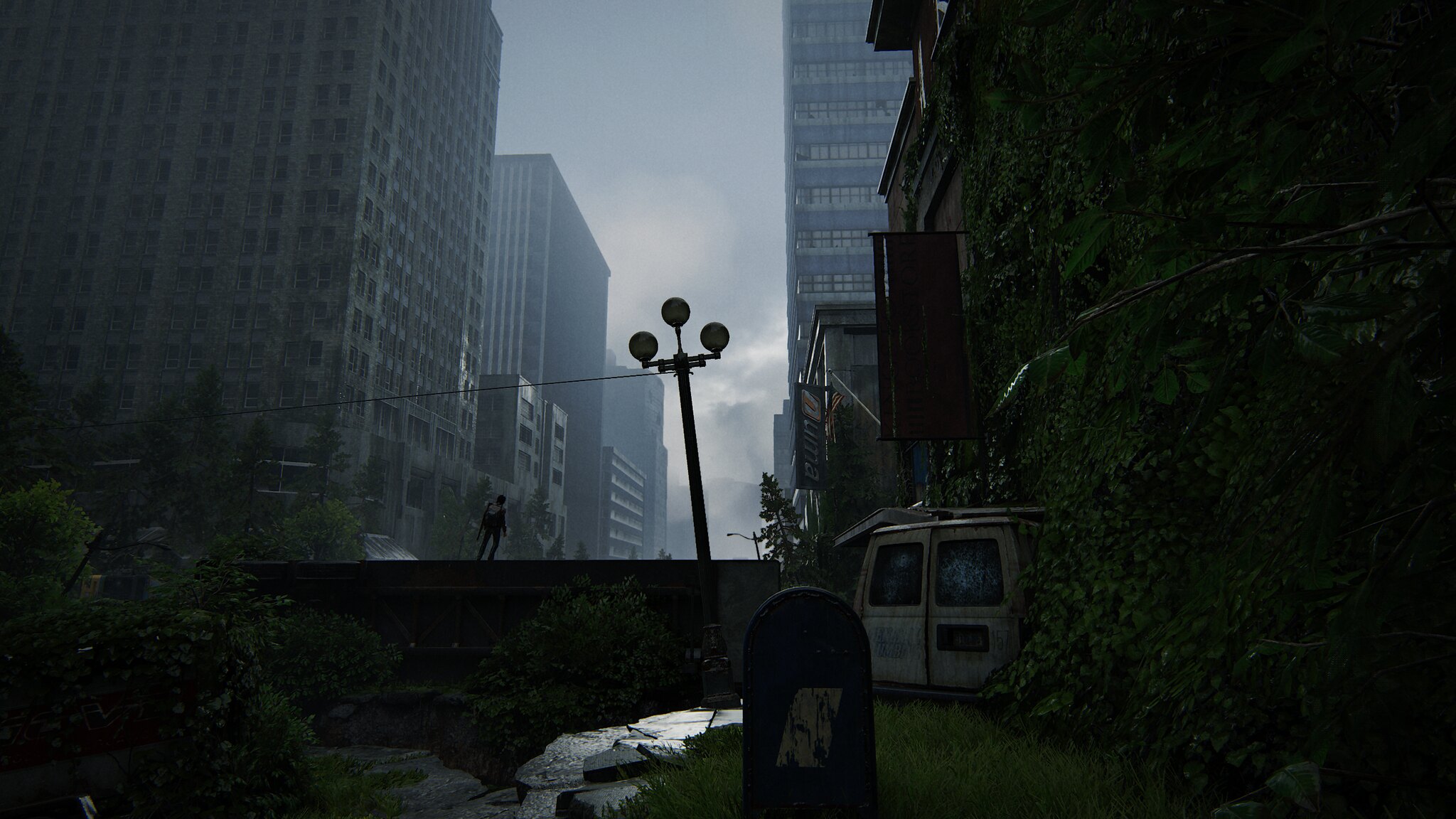This highly detailed and crisp image, reminiscent of a high-quality video game scene in 4K resolution, captures a compelling urban cityscape. Dominating the foreground is a van that has collided with a wall, creating a sense of dramatic tension. Nearby, a blue public mailbox stands as a quiet sentinel amidst the chaos, ready for daily mail pickups. In the background, under the cover of darkness, the silhouette of a lone figure can be seen standing resolutely in the middle of a deserted street. Towering buildings encircle the scene, contributing to the eerie, almost post-apocalyptic atmosphere of the city.